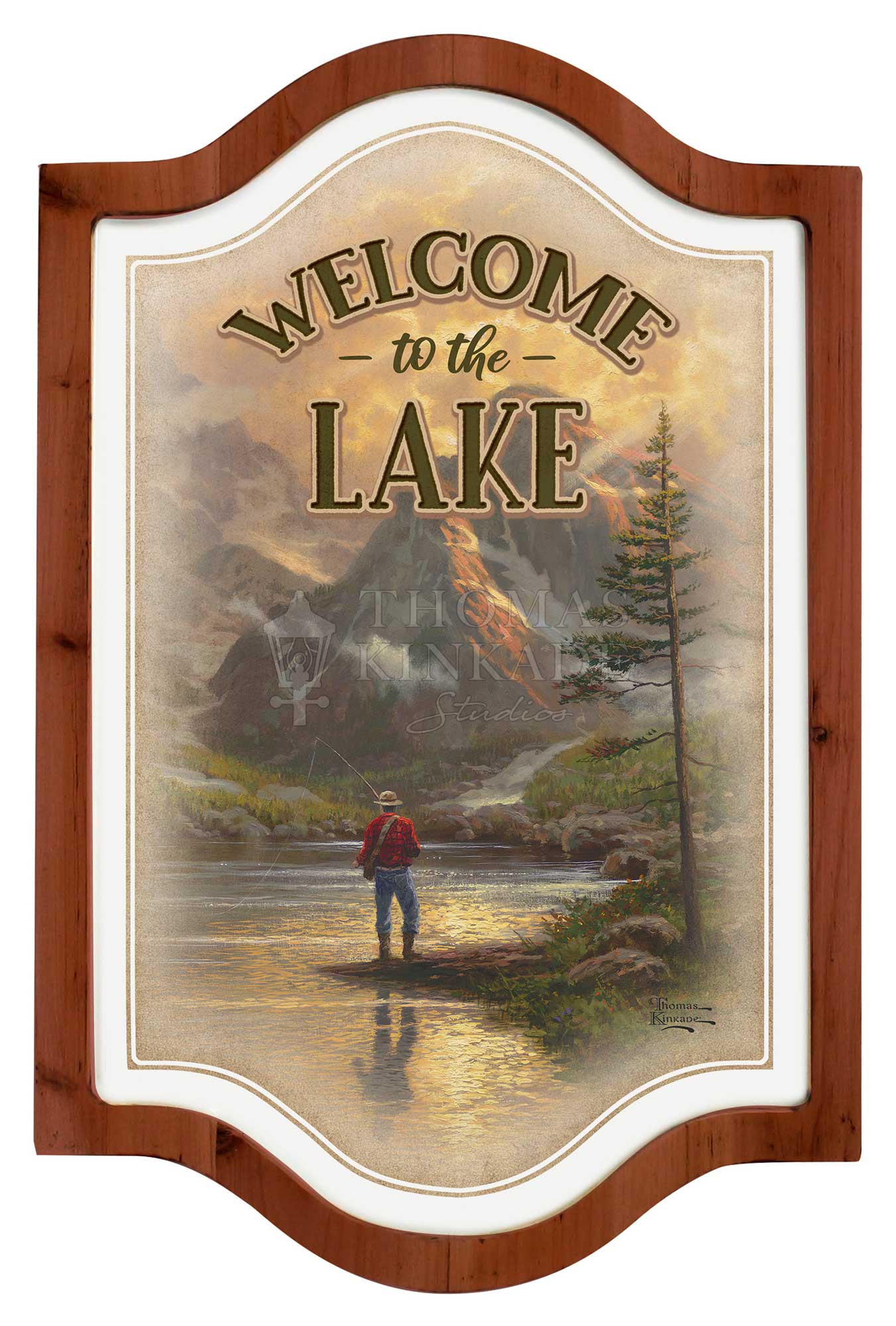This decorative plaque features an inviting "Welcome to the Lake" message, making it a perfect addition to a lake house. The design presents a harmonious mix of rustic and elegant elements. The sign is framed with a natural woodcut border, followed by a sequence of borders: an inner white border, a thinner gold border, another white border, and a final thin delineation around the main image. The entire design is shape-cut, contributing to its distinctive aesthetic.

At the top of the sign, the words "Welcome to the Lake" are written in a cheerful, curving font, with the phrases "to the" placed centrally between "Welcome" and "Lake." Below this text, the illustration features a man standing at the edge of a serene lake or riverbank. Dressed in a red shirt, fishing boots, and a fishing hat, he is engrossed in fishing, holding a rod that is already cast into the water. Beside him stands a lone, young, and slender tree with minimal foliage, adding a touch of simplicity to the scene. The backdrop is completed with a range of majestic mountains, adding depth and tranquility to the image.

Subtly woven into the artwork, a transparent watermark suggests the claim of the artist or the entity that owns the rights to this image. Additionally, the artist's signature can be found in the bottom right corner of the painting, though it is small and unobtrusive. This detailed and charming depiction captures the essence of a peaceful lakeside retreat.